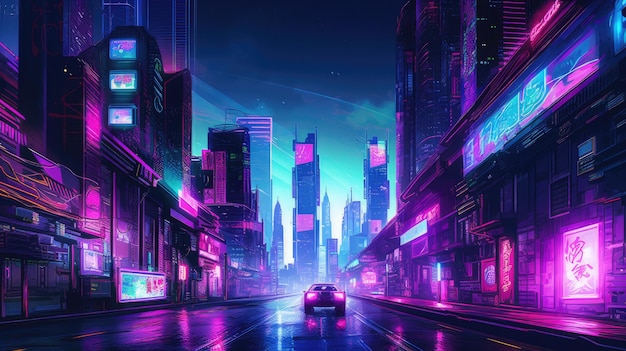The image showcases a vibrant, futuristic nightlife in a sprawling cityscape. Tall buildings dominate both sides of the scene, with towering skyscrapers visible in the distance. Central to the picture is a car driving towards the distant buildings, its illuminated taillights gleaming. The entire scene is awash in vivid, dazzling neon lights—in hues of purple, blue, pink, and blue—emphasizing the nightlife atmosphere. The wet road reflects these neon signs, adding to the spectacle. The sky above is a dark bluish-green, contrasting with the vividly colored cityscape below. The overall palette of the image is dominated by striking neon pinks, lending the scene an otherworldly glow.